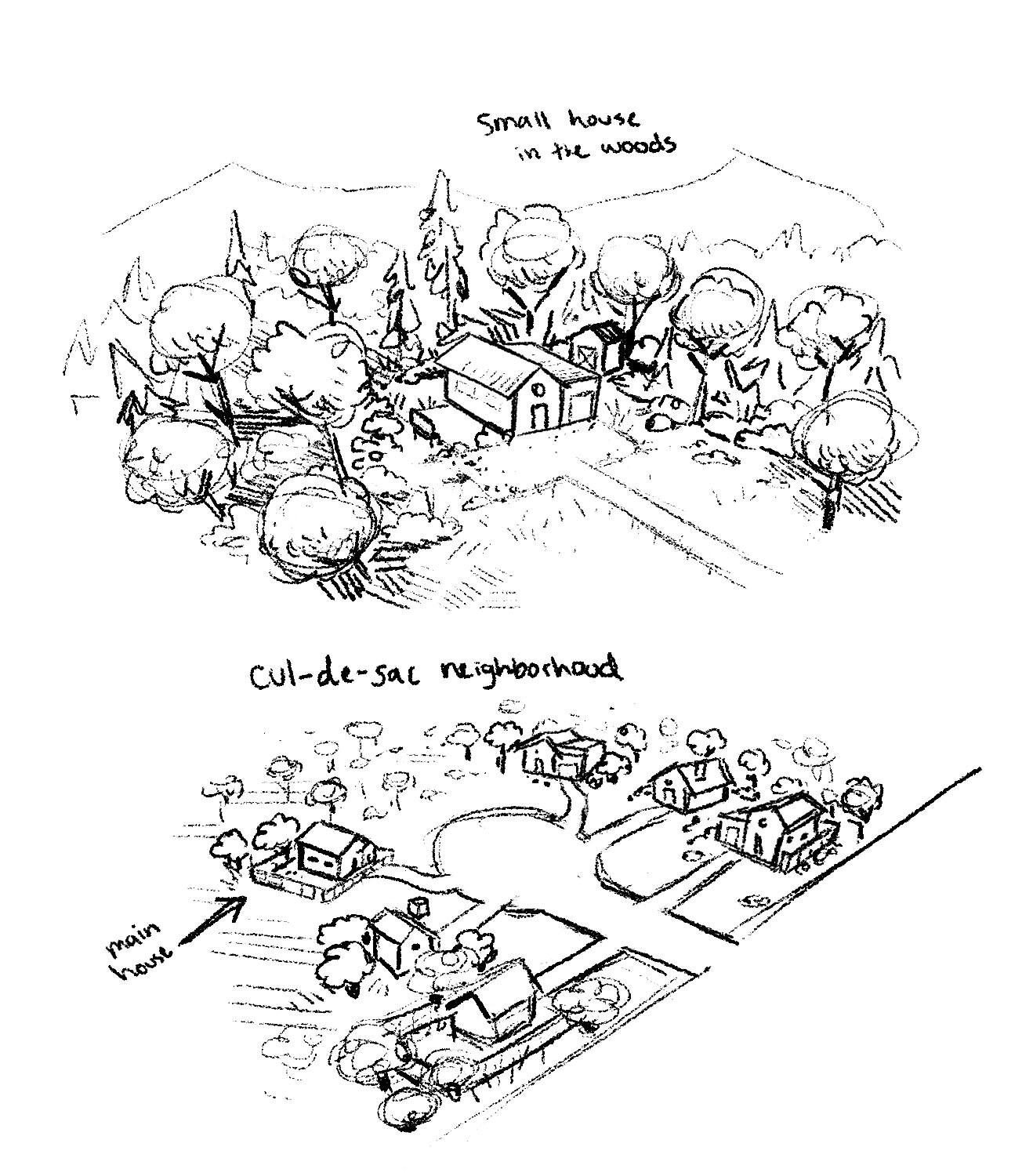This black-and-white illustration features two sketched sections of what appear to be interconnected neighborhood layouts. The top half of the image is labeled "small house in the woods" and highlights a secluded home surrounded by a dense forest of various types of trees and low-lying mountains in the background. The house itself is modest, with a single door, a pitched roof, and a small window above the door. A walking path or driveway leads to the front of the house, which sits next to a tool shed.

The bottom half of the illustration is labeled "cul-de-sac neighborhood" and depicts a suburban area from a bird's-eye view. This section includes a cul-de-sac with six houses, each with driveways extending from the main road. One house, pointed out by an arrow, is labeled "main house." Trees are dotted around the neighborhood, and some houses have fenced-in yards and garages. Occasional details like smoke coming out of chimneys add a touch of life to this suburban scene.